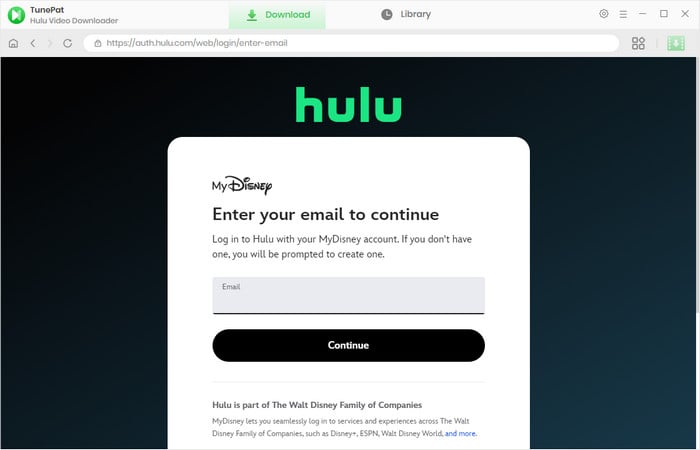The image displays the login screen for the ToonPad Hulu Video Downloader application. Prominently featured in the top-left corner is the ToonPad logo. Just below the application header, the Hulu logo is visible, indicating the service the application supports. The login section contains clearly labeled fields for "Email" and "Password," with respective input boxes beneath each label. A clickable link for "Forgot Password or Email?" is provided for user assistance. Below the input fields is a gray "Login" button. The overall layout is clean and minimalist, featuring a white background and black text for optimal readability. The login fields and button are centrally aligned within the main content area, emphasizing simplicity and ease of use. However, the legal standing of using such an application remains ambiguous; although it allows users to download content they have access to, questions linger about the legality of downloading for future viewing once a subscription ends. This issue is further complicated by evolving laws, particularly in the context of AI advancements.